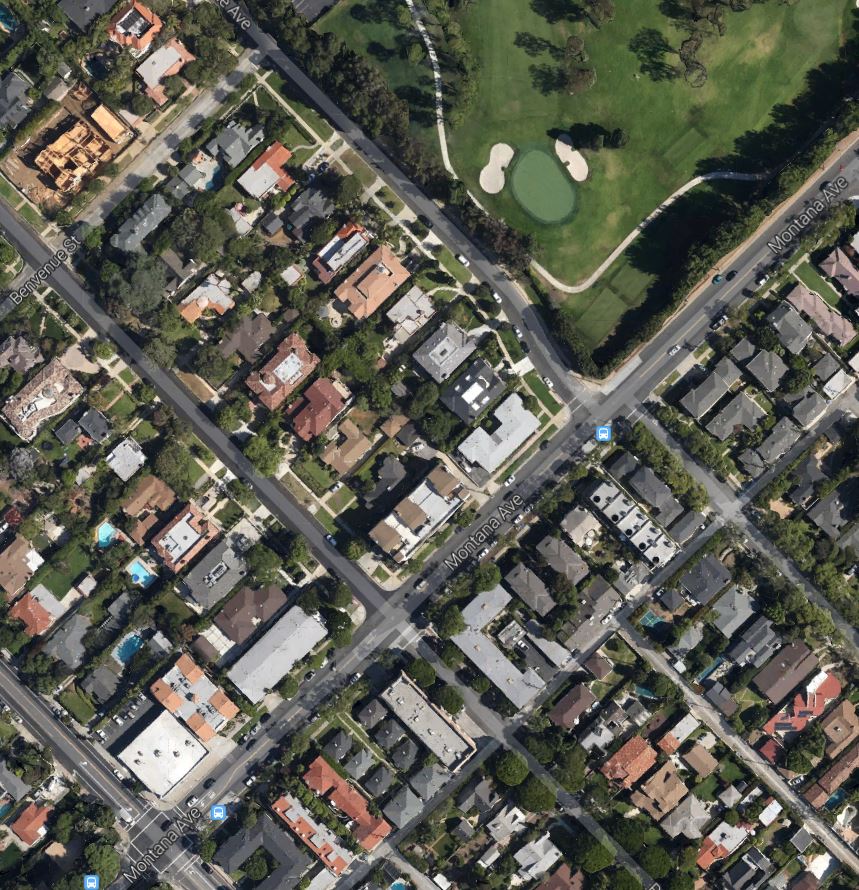Aerial view showcasing a residential neighborhood with a diverse array of houses. Roofs vary in color, with some being tan and others in shades of gray, including very dark gray. Many backyards feature swimming pools. In the upper right corner, there is a large grassy field, with a green pond at its center, flanked by two light-colored circular areas that could be sandy patches, suggesting a potential golf course. A long white path traverses the field, likely serving as a walking trail or part of the golf course. Streets weave through the neighborhood, fronting the houses and their yards. Tiny, almost indistinguishable figures—possibly cars or people—can be seen. Near the center, at the back of a house adjacent to the grassy area, there's a small blue square with a white car icon, enhancing the detailed landscape.